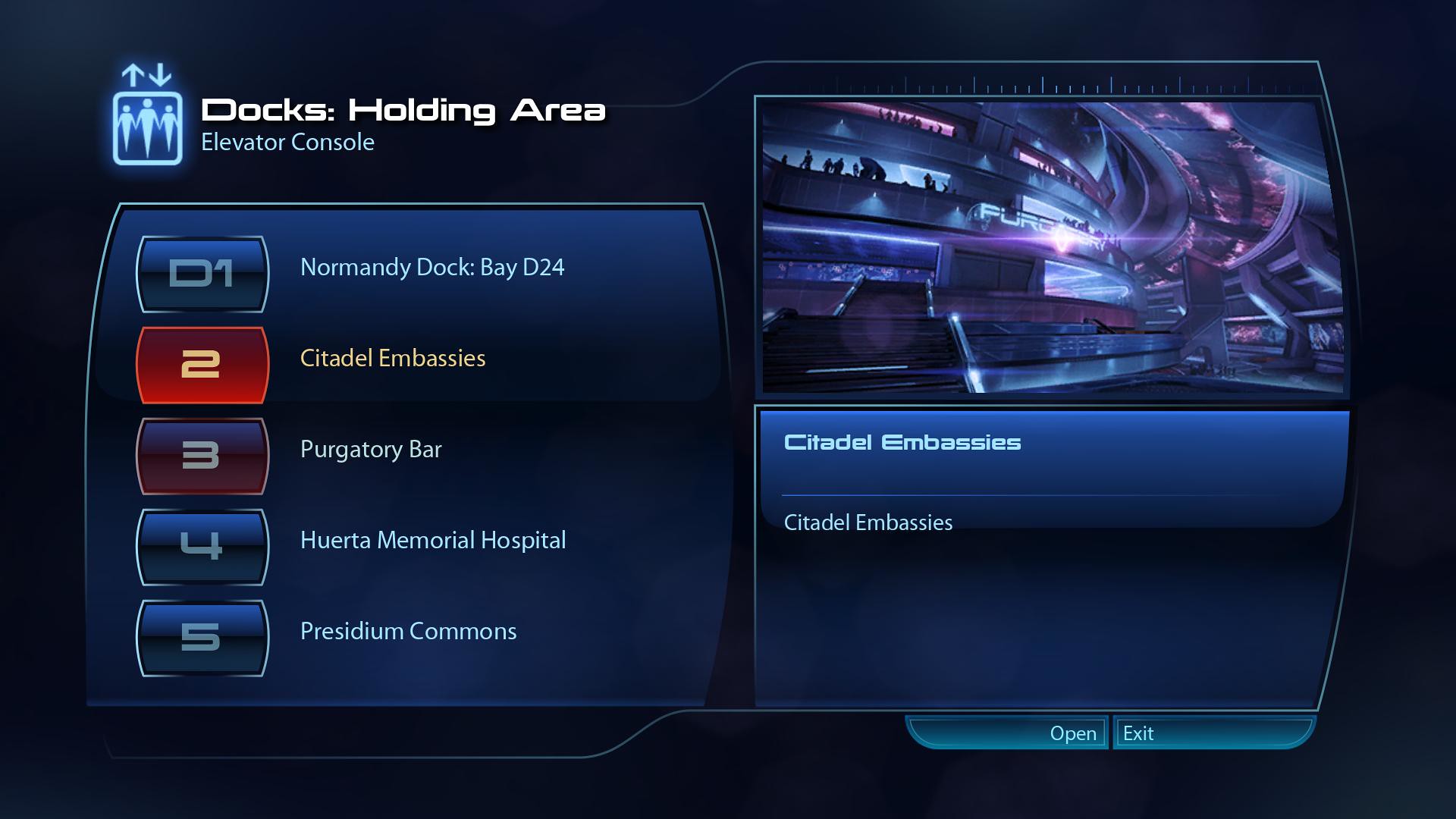This image appears to be a screen capture from a futuristic online video game, featuring an in-game menu. The layout is set against a predominantly black and dark blue digital interface. In the upper left corner, there's a light blue square emblem containing three white stick figures and up and down arrows. Next to this emblem, in white text, are the labels "Dock’s Holding Area" and "Elevator Console." Below these labels is a vertical list of five destinations, each associated with a numbered button:

1. Normandy Dock Bay D24 (D1)
2. Citadel Embassies (2)
3. Purgatory Bar (3)
4. Huerta Memorial Hospital (4)
5. Presidium Commons (5)

To the right of the list, the screen expands into a larger, almost rectangular window displaying a CGI-rendered image of a futuristic, multi-level space station or mall. This station is characterized by rounded walls in shades of dark blue, purple, and silver, with a central cylindrical concourse populated by small human figures. Below this CGI image, "Citadel Embassies" is written twice in descending font size. At the bottom right of the screen, there are two green button tabs labeled "Open" and "Exit," which hint at interactable options within the game. The overall aesthetic of the menu combines sleek, modern design elements with a distinctly sci-fi atmosphere.